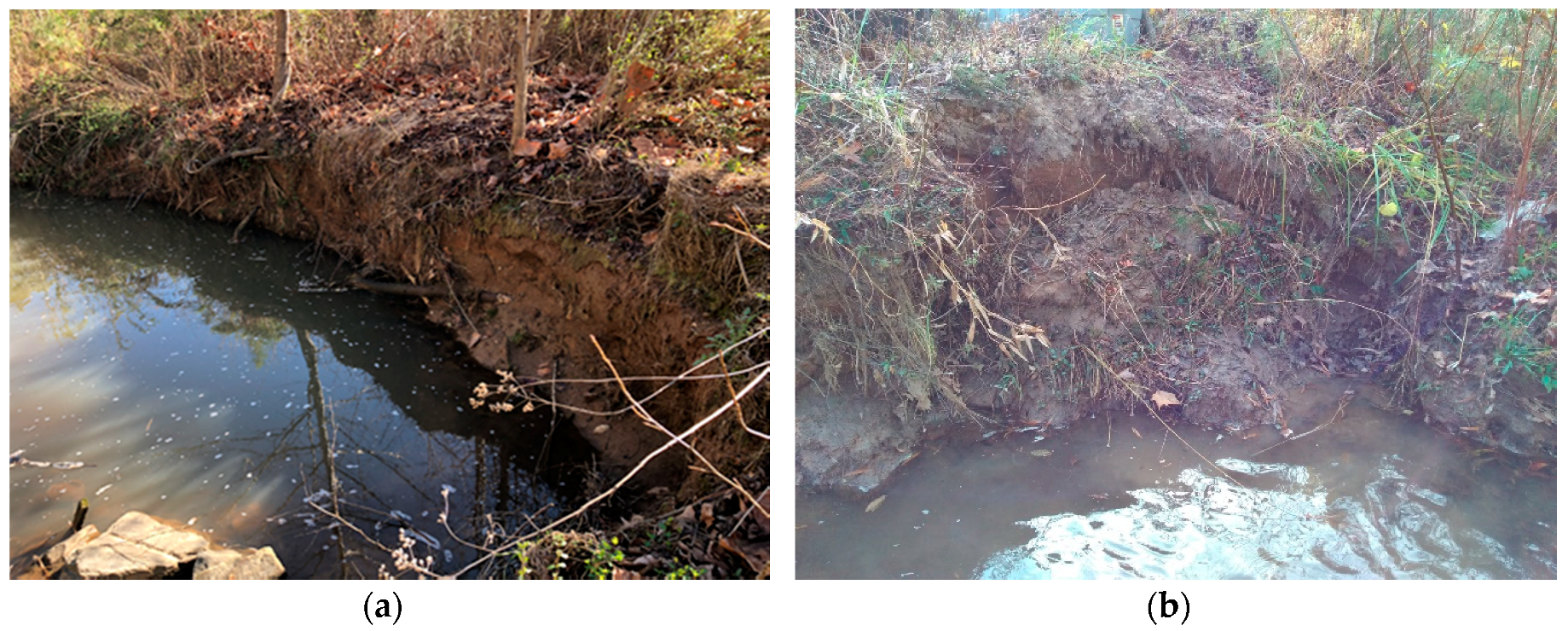The image is a side-by-side comparison of two different parts of the same stream or river, labeled (a) and (b) in lowercase parentheses beneath each section. The left image (a) is more brightly colored and depicts the edge of a muddy riverbank with a body of water visible. The water has a slight white speckled matter on its surface, and there is a rock or possibly trash in the bottom right corner of the image. The banks have grassy areas and twigs extending from the edge. The right image (b) shows a darker, more eroded riverbank with fallen grass and foliage leaning into a muddy and duller-colored waterway. The vegetation is more abundant and disorganized, suggesting a more degraded state, which could indicate different stages or impacts on the ecosystem of the stream. Both banks in image (b) are less smooth and have visible ripples on the water surface.